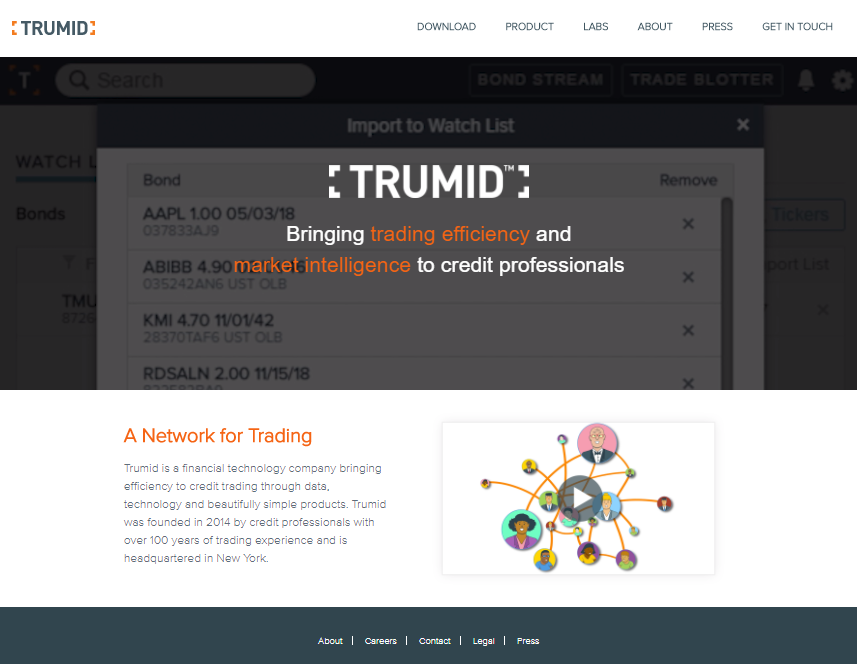A detailed caption for the image could be:

The image depicts a webpage with a predominantly dark theme. At the top left, the background is white, with subtle orange markings surrounding the word "TRUMID." The logo "TRUMID" is prominently displayed in blue. 

Towards the top right middle section of the page, a navigation menu with light blue links reads "Download," "Product," "Labs," "About," "Press," and "Get in Touch," extending from the center to the right edge of the page.

The main section of the page appears dim, likely due to an overlay that needs to be clicked off to reveal the content behind it fully. In the center of this darker overlay, the TRUMID logo is displayed again in white, flanked by orange markings. Below the logo, the phrases "Bringing Trading Efficiency" and "Market Intelligence" appear in a combination of white and orange text, followed by "to Credit Professionals" in white, set against the middle of the page over a backdrop showing faint numbers and columns.

Further down on the page, an orange-highlighted phrase on a white background reads "A Network for Trading," followed by detailed information about the company. To the right, a white rectangle contains a series of images of people, with arrows indicating navigation between images. A central play button, represented by a gray oval with a white arrow, suggests the presence of an interactive video.

At the bottom of the page, a dark gray or blue banner stretches horizontally with white text links reading "About," "Careers," "Contact," "Legal," and "Press," each separated by vertical lines.